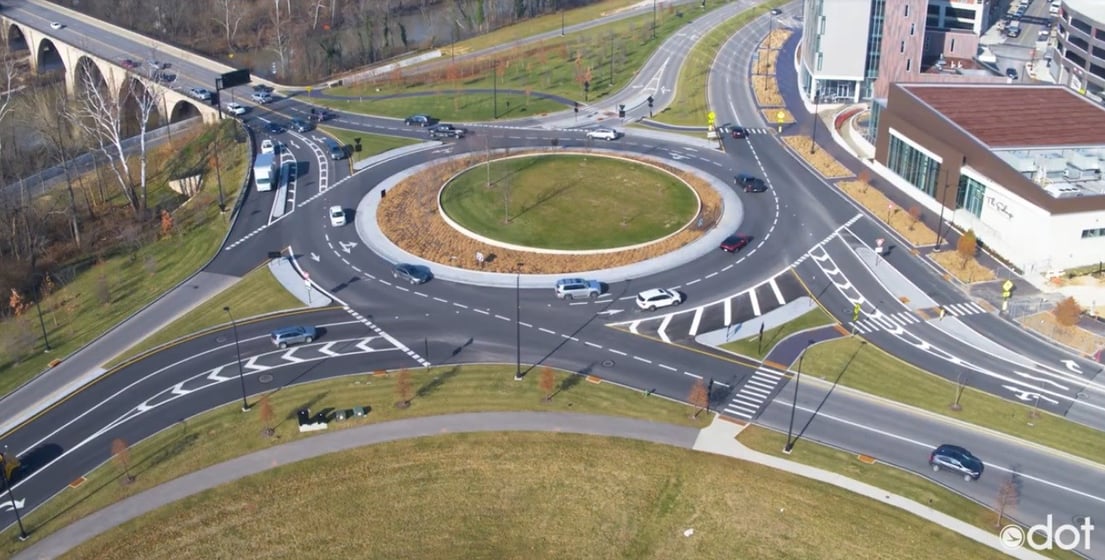This horizontal rectangular color aerial photo captures a bustling suburban roundabout surrounded by various urban features. The central island of the roundabout features a circular grassy area bordered by a brown, dirt-like zone, indicative of either fall foliage or dry conditions. The roundabout efficiently manages traffic with its four major streets, each contributing two lanes in both directions, making a total of eight lanes flowing in and out.

On the right side of the image, several buildings are visible, including what seems to be a low building that might be a restaurant and adjacent apartment buildings of varying heights. The bottom of the image shows a grassy area intersected by a sidewalk that curves towards the lower right.

Notably, in the upper left corner of the frame, there's a bridge resembling an aqueduct with long stone archways, spanning over what could be a railway. The bridge facilitates traffic into the roundabout and is accompanied by numerous vehicles, including a noticeable large truck. The roadways of the roundabout are a stark dark gray, contrasting with the dried-out grass surrounding it.

In the lower right corner, the text "DOT" is visible, although its significance is unclear. The overall scene is dynamic with multiple cars navigating the roundabout, particularly from the bridge entrance, indicating a central hub of transportation amidst a suburban setting.